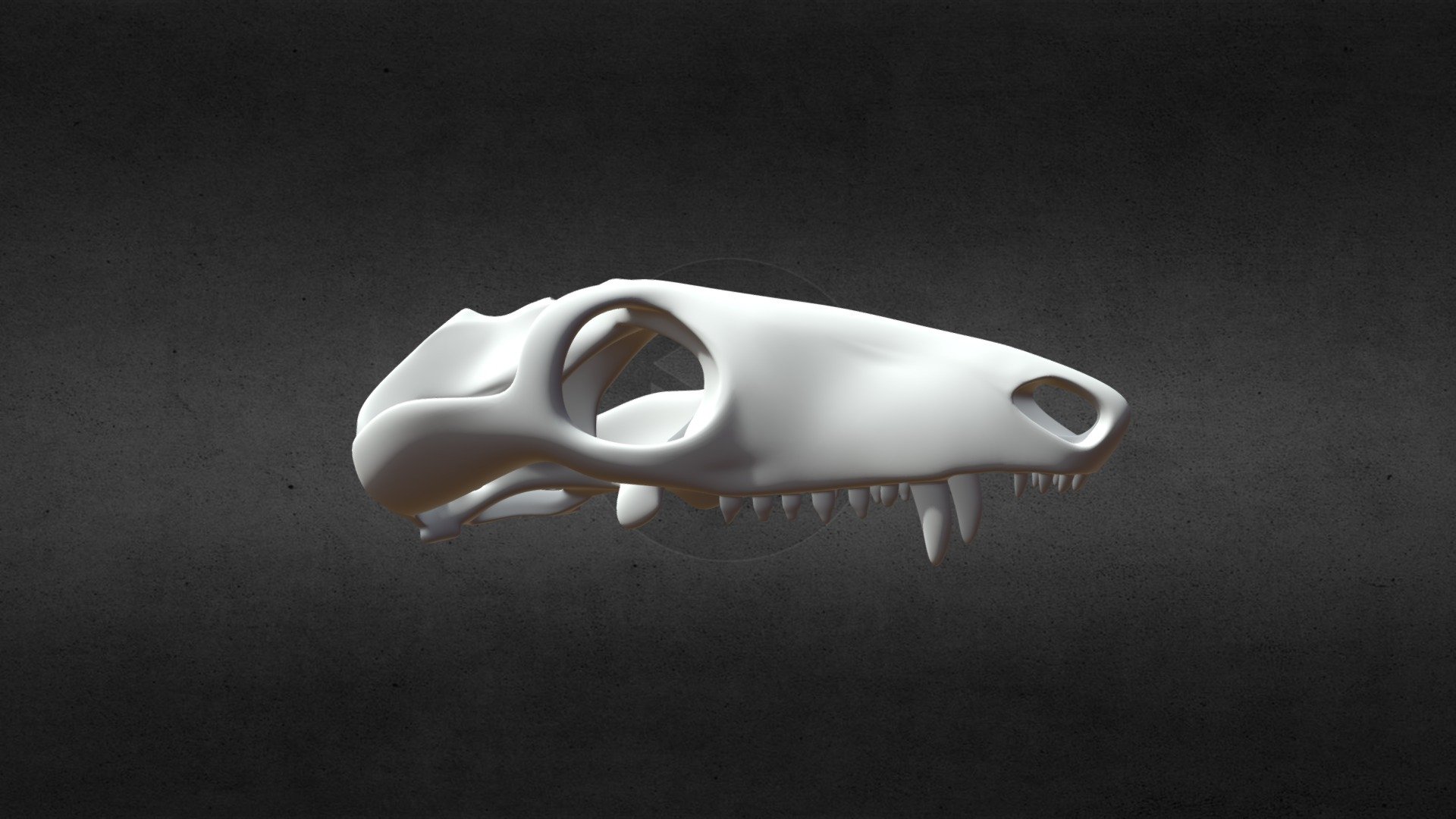The image depicts a digitally rendered side profile of an animal's upper skull, characterized by its notably elongated horizontal structure. Centered within the image, the skull displays a detailed anatomy including prominent features such as large nasal holes positioned towards the right. The eye socket, situated slightly to the left of center, leads into the extended snout area where the nostrils are located. Below the eye socket and extending to the right, a row of teeth is visible, featuring two large fangs set back from the front, surrounded by smaller, needle-like teeth, and culminating in a significant molar at the rear. The entire skull is rendered in shades of white, brown, gray, and black against a gradient gray background. A small circular detail is positioned behind the skull, adding to the intricate digital representation seen in the image.